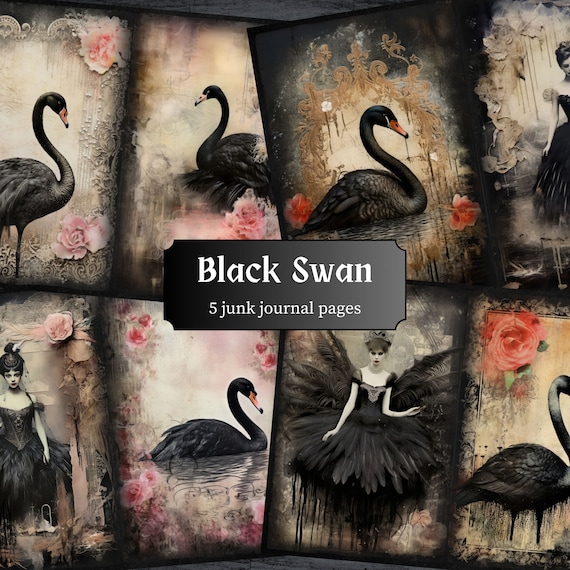The cover page of the Black Swan journal features a meticulously arranged collage of images depicting five black swans and three women, all of which are enveloped in a dark, Gothic aesthetic. The composition of the page is neatly divided into eight sections - four on the top row and four on the bottom row. In the top row, three black swans are positioned from left to right, followed by an image of a woman in a black dress and hat. The bottom row mirrors this pattern but starts with a woman dressed in a dark, Gothic boudoir or ballet attire with feathered wings, followed by a black swan, another woman in a similar dark ensemble, and lastly a black swan. The backdrop of these images is heavily faded, with whites, grays, purples, and pinks bleeding through, enhancing the vintage and eerie aesthetic. Gold and pink accents, frilly designs, and flowers adorn the edges, adding a delicate yet dark contrast to the overall dark color palette. In the center of the cover, a black box with white lettering prominently reads "Black Swan, five junk journal pages," potentially indicating that the image was AI-generated or created with an art program.